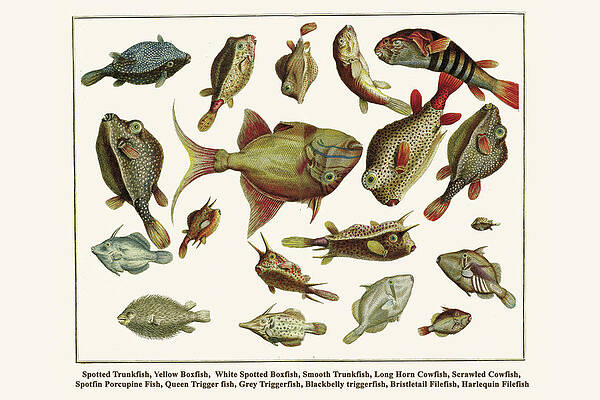The image is a rectangular, horizontally oriented illustration resembling a piece of paper against a beige background. At its center is a thin black border framing a scientific-style diagram of various fish species. The fish, presented in a manner reminiscent of a classification book, are illustrated in colored pencils or inks showcasing a diverse palette including green, beige, blue, and reddish hues. Each fish appears in different poses—some looking up, others down or to the sides—giving a sense of dynamic placement. Below the illustrations, black text labels the species: Spotted Trunkfish, Yellow Boxfish, White Spotted Boxfish, Smooth Trunkfish, Longhorn Cowfish, Scrawled Cowfish, Spotfin Porcupinefish, Queen Triggerfish, Gray Triggerfish, Black Belly Triggerfish, Bristletail Filefish, and Harlequin Filefish. The fish feature speckled scales and appear visually similar, with discernible fins and eyes, yet there are no numerical or alphabetical markers linking each illustration to its corresponding name.